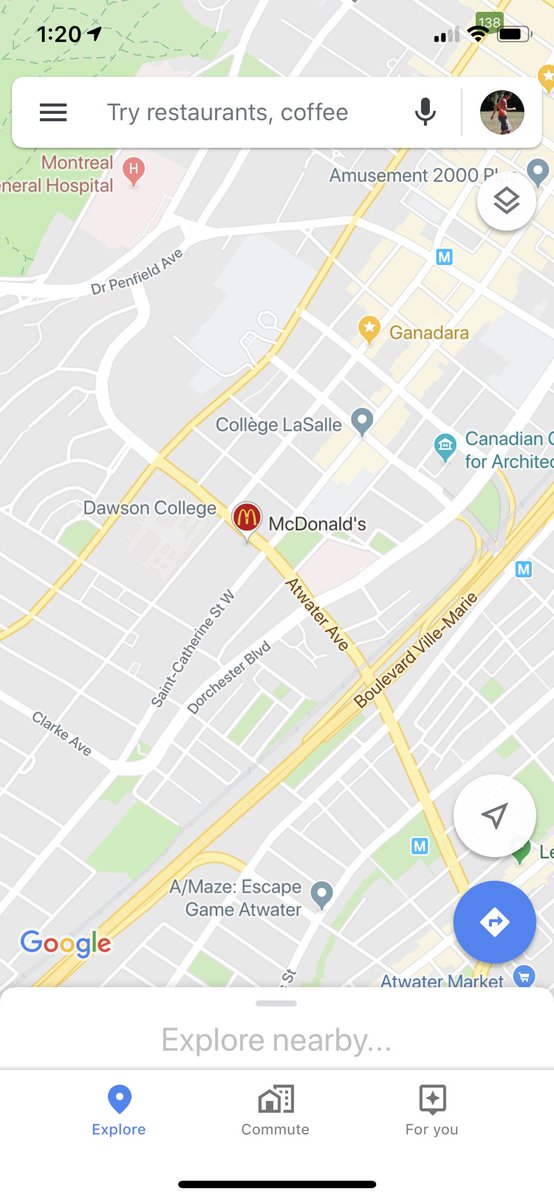This image is a screenshot of a Google Maps interface on a smartphone, depicting a section of an unspecified city. The phone displays the time in the top-left corner as 1:20, with indicators for Wi-Fi connection and battery status. Dominating the top of the screen is a search bar with the prompt "Try restaurants and coffee," accompanied by a circular user avatar and a microphone icon for voice search.

The map itself presents a detailed overview, featuring a network of streets, highways, and names of surrounding areas. A notable point on the map is marked by a bright orange-yellow pin indicating "Ganadara." To the left, a pink "H" icon denotes the Montreal General Hospital, situated near a McDonald's restaurant.

The map also highlights two educational institutions: College LaSalle and Dawson College, both located on the western side of the area displayed. The main thoroughfare running through the map is identified as Boulevard Ville-Marie.

In the bottom-right corner, there is an option labeled "Explore Nearby," alongside three icons offering further functionalities: "Explore," "Commute," and "For You." A black bar spans the very bottom of the screen, encapsulating these navigational choices.